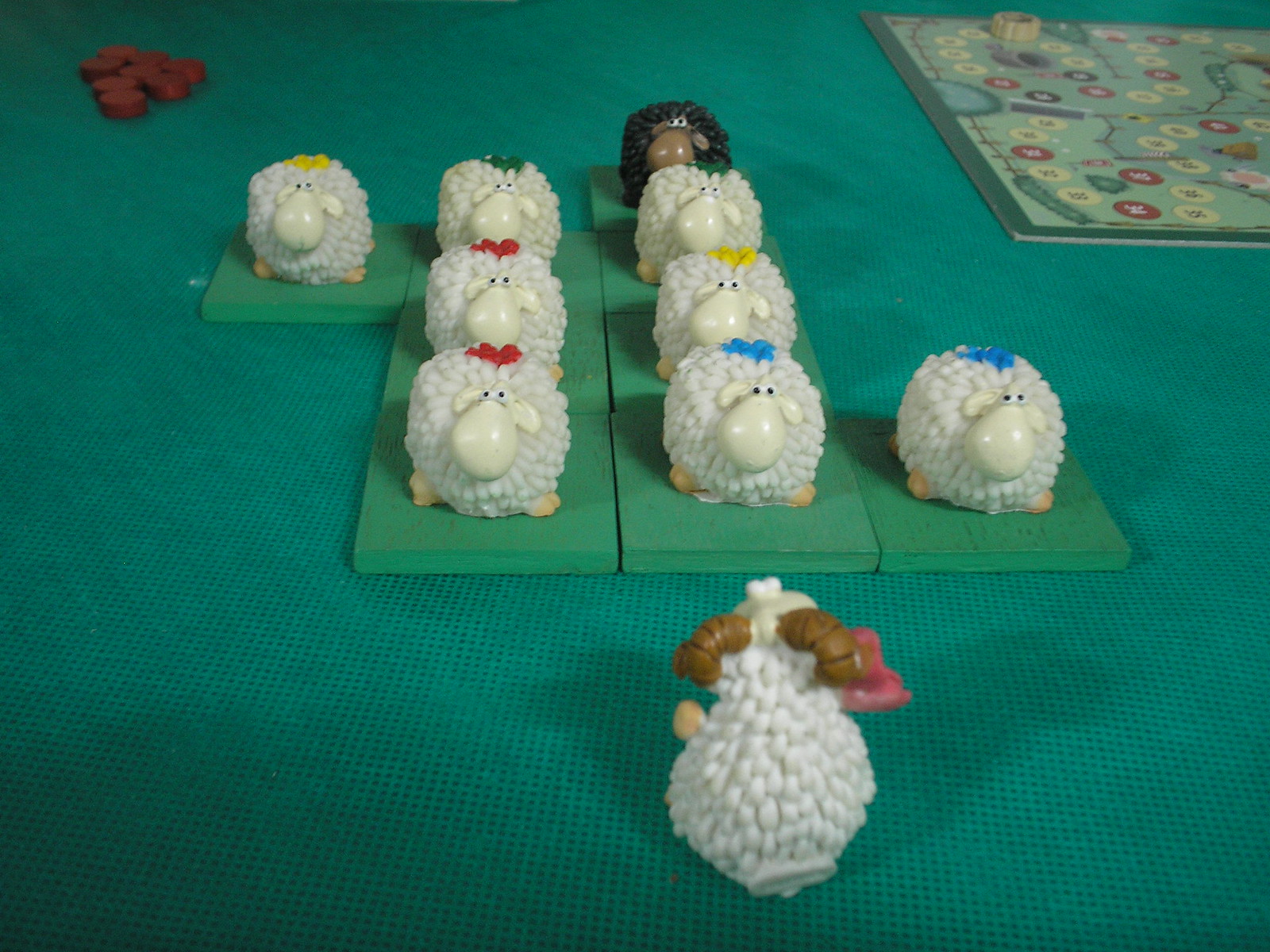This photograph captures a unique gaming table setup viewed from an angle, showcasing a whimsical scene of handmade toy sheep arranged as if in a classroom or gathering. The table is covered with a textured, emerald-green cloth, creating a vibrant backdrop. 

In the middle foreground stands a lone ram with brown horns and a fluffy white body, seemingly made of plastic or rubber. This ram faces a structured arrangement of nine other sheep, all positioned on thick, green square bases, looking outward from the scene.

These nine sheep vary in color and decoration: eight are white, adorned with different colored markings or tiny hats in blue, green, red, and yellow, while the one at the very back is distinctively black with a brown nose. 

The top right of the image features a game board with a bluish-green trim decorated with red, white, and green circles, suggesting pathways or spaces for game pieces. In the top left corner, a stack of copper-colored counters or tokens, possibly used for a board game, adds a splash of metallic sheen to the tableau. The overall image blends elements of playful creativity with a hint of organized gaming.